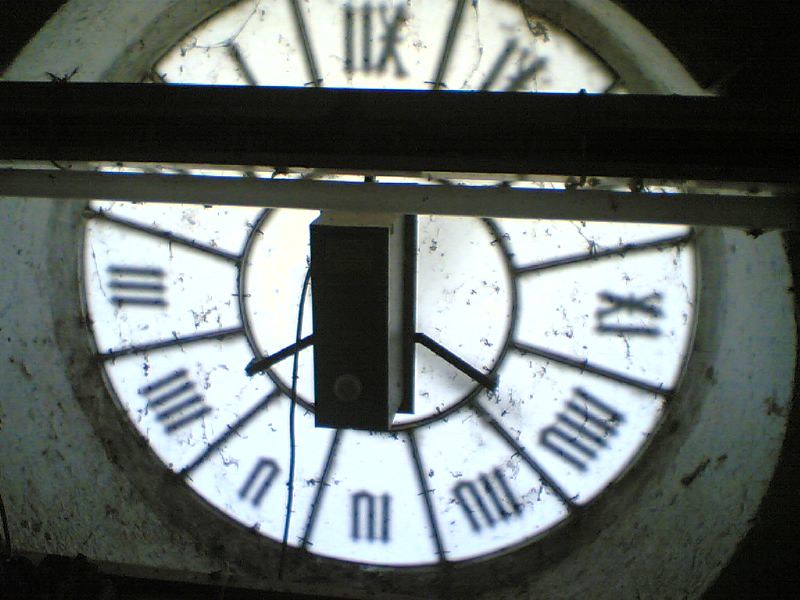The photograph appears to be taken through a smudged and dirty window, with numerous specks of dirt visible across the glass. Dominating the foreground is an unspecified mounted object, possibly a light fixture or holder, which seems to rest directly on the glass. Beyond this object stands a white clock with black Roman numerals, though the numbers at the top are partially obscured by the foreground fixture. The area surrounding the clock is a murky gray, and each of the four corners of the image is black, adding to the overall sense of disorientation. The image is quite blurry, making it difficult to discern the exact perspective or additional details. The only identifiable element is the clock, but even this is shrouded in fuzziness.